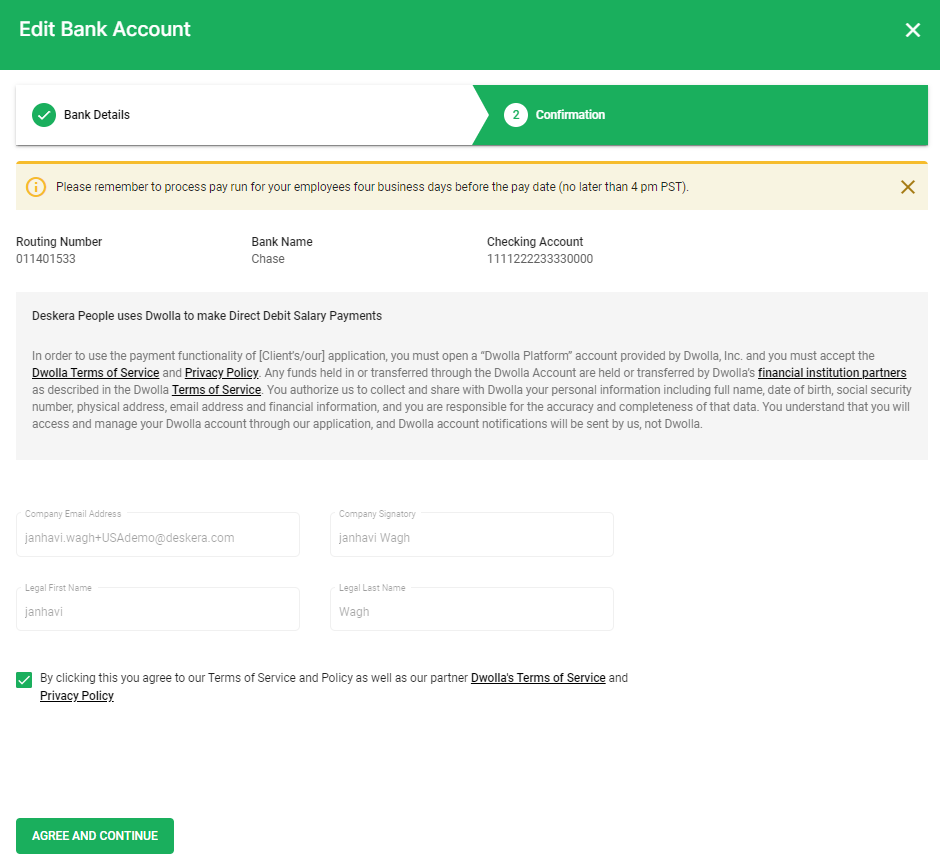In this image, we are looking at a detailed screenshot of a website interface for editing bank account details. At the top, there is a green header with white text on the left side that reads "Edit Bank Account." Below the header is a divided block: the left side is white and labeled "Bank Details" with a green circle containing a white checkmark, while the right side is green with a white circle featuring the green number "2" labeled "Confirmation."

Separating these sections is a gold line running horizontally across the screen. Below this line, there is a yellow circle on the left side with an eye icon in its center. Next to this circle is a reminder in black text: "Please remember to process pay run for your employees 4 business days before the pay date, no later than 4 p.m. PST."

Further down, on a white background, black text provides specific bank account details: "Routing Number: 011401533, Bank Name: Chase, Checking Account: 111122223333000." At the bottom, set against a gray background, a bold black text states, "Descara people use DWOLA to make direct debit salary payments."